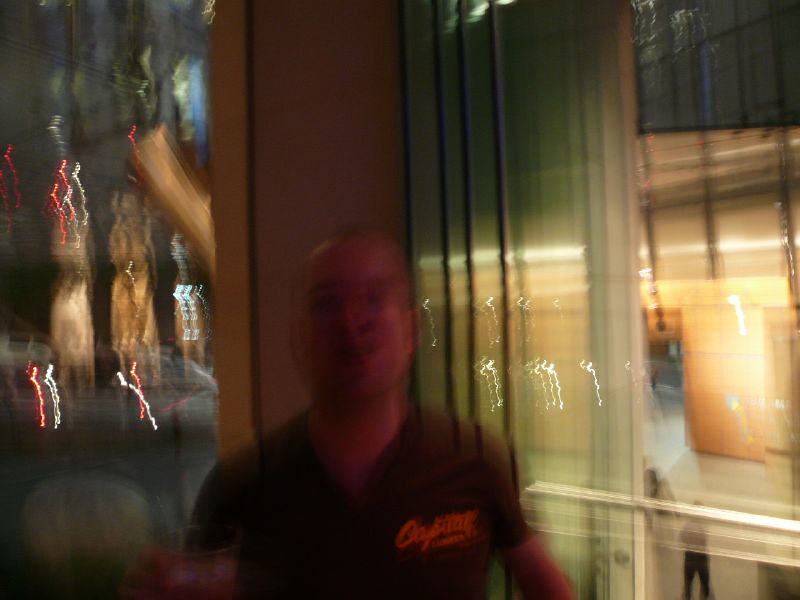This color photograph features a dimly lit scene with noticeable motion blur, making finer details hard to distinguish. At the center of the image is a man, whose head and torso are visible. He is wearing a dark t-shirt adorned with an unreadable orange logo on the left breast. To his right, a blurry streetscape comes into view, adorned with what seem to be trees and street lights, their forms elongated into streaks of red and white light, likely due to the camera motion. This gives an impression of bustling urban activity. A tall brown pillar stands behind him, directing the viewer's gaze towards the right, where the windows of a building can be seen. These windows are partially illuminated, with indistinct figures moving inside. The windows just behind the man's left shoulder have a dark green hue, possibly due to blinds, while the other windows appear more transparent, offering a glimpse into the interior lights and activity.